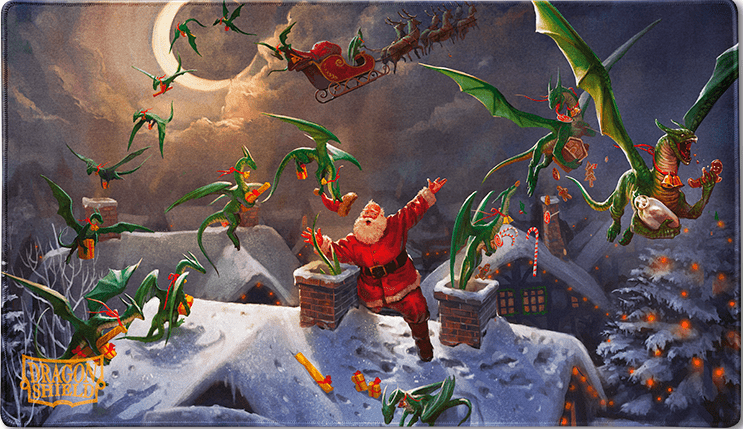The image is a vibrant, snowy holiday scene featuring a snow-covered house with a prominent double chimney. Santa Claus, notably without his hat, is depicted on the rooftop in a precarious position, as if he is slipping. Surrounding him, scattered presents rest on the snow-covered roof, hinting at a sudden mishap. Santa's sleigh, now commandeered by eerie, dragon-like creatures, soars through the gray, cloud-filled sky, with the moon—more specifically, a quarter moon—glowing faintly in the background. The creatures, known as Dragon Shield, have ominously stolen Santa's sleigh and its cargo, including toys and children. Footprints mark Santa's path on the snowy roof, indicating his struggle. Adding to the festive scene, Christmas lights adorn the trees and house, casting a warm glow on this chaotic but magical night.